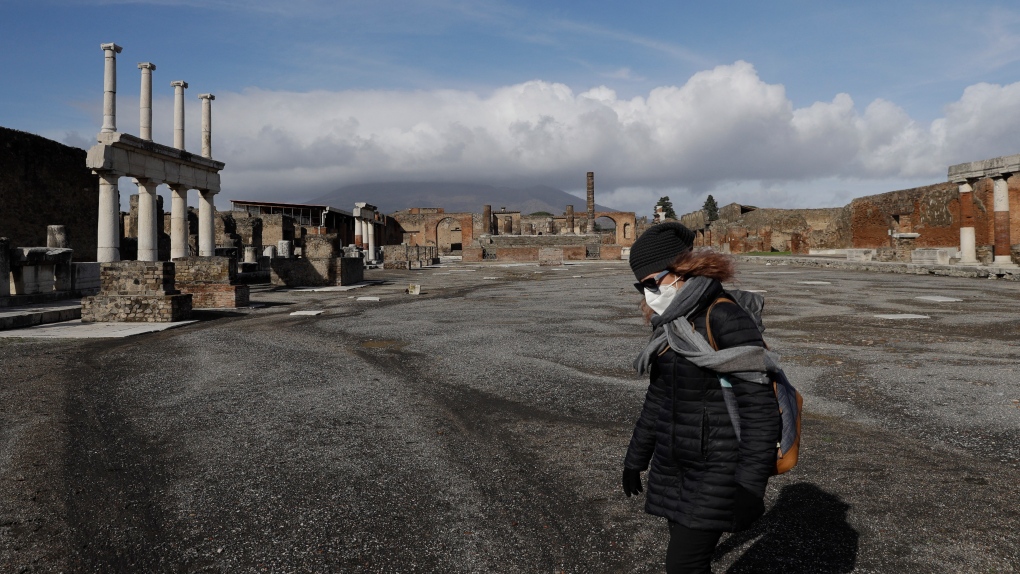In the foreground of the image, a woman is walking on a pebble-strewn path, dressed in a black puffy winter jacket and black pants. She has a gray scarf wrapped around her neck and a white mask covering her face. Her outfit is completed with black gloves, a black beret, and black sunglasses that have a bluish tint on the arms. Slung over her left shoulder is a dark gray bag with brown accents at the bottom and on the straps. Her brown hair peeks out from under her beret as she looks downward.

The scene around her appears to be a mix of old and modern remnants, creating an abandoned complex atmosphere. To her left, the ruins of what looks like a Greek column facade evoke the grandeur of an ancient coliseum. In contrast, off to the right, there are what seem to be abandoned brick buildings with pillars and arched entrances. The road she walks on is shaded with hues of gray, white, and black. In the distant background, a range of mountains partially shrouded by clouds looms under a blue sky. An unusual chimney-like structure stands in front of the mountains, adding to the eclectic mix of the scene. The woman’s shadow is cast behind her, accentuating her movement towards the left of the image.